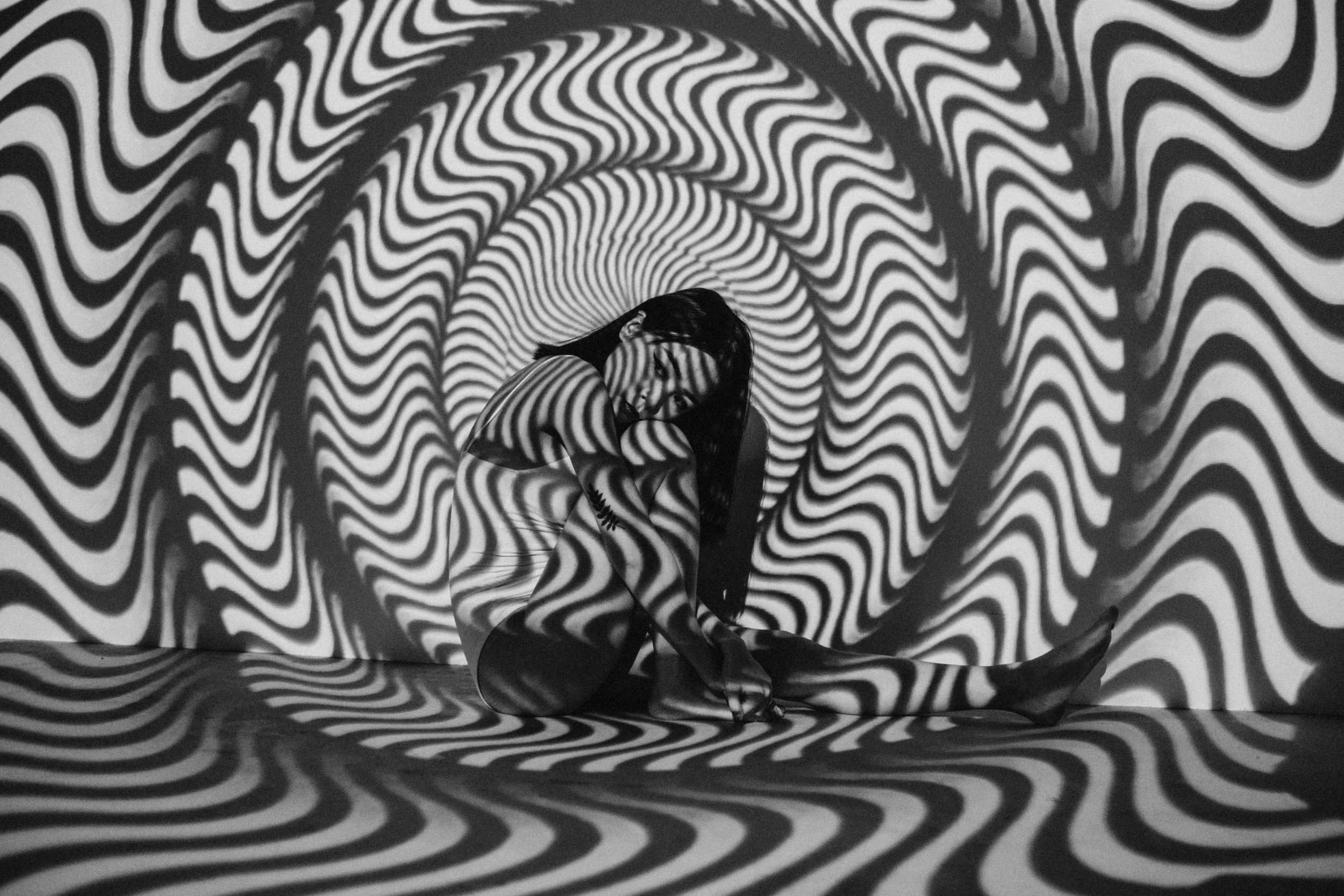The photo features a female model, seated calmly in the center of a mind-bending, warping tunnel that embodies a kaleidoscope effect of black and white waves. The tunnel's swirling lines, resembling zebra stripes, envelop her completely. She has medium-length black hair resting her head on her hand in a pensive manner. The model appears to be Asian and is wearing a white leotard, with no shoes and a prominent leaf tattoo on her right forearm. Her eye makeup is elongated, and she gazes forlornly into the left corner of the frame. The photo, characterized by its stark black and white palette, contains no text or other objects, focusing solely on the solitary figure amidst the wavy, hypnotic patterns, suggestive of a high-fashion modeling shoot.